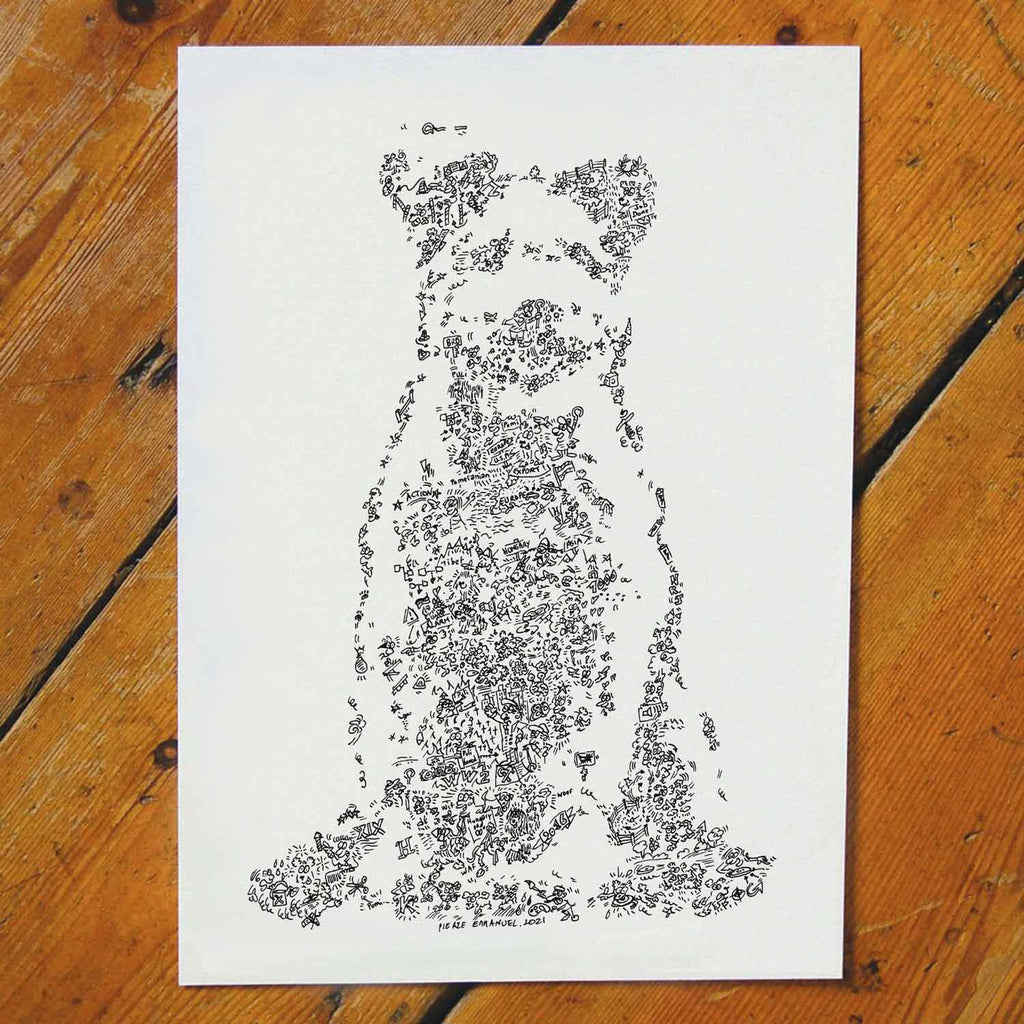This color photograph depicts a unique hand-drawn illustration of a dog, meticulously composed using words and symbols instead of traditional lines. The dog, identified as a "Pubey," is shown in a sitting position, rendered in black ink on a white rectangular sheet of paper. The dog features pointy ears, discernible eyes, and a defined mouth, with text artfully arranged to form the shape of its body, including its paws. The paper rests on a brown wooden surface, likely a picnic table or a wooden floor, distinguished by visible cracks. The illustration, executed in a style resembling pointillism, bears an illegible signature at the bottom, possibly reading "Emmanuel 2021."